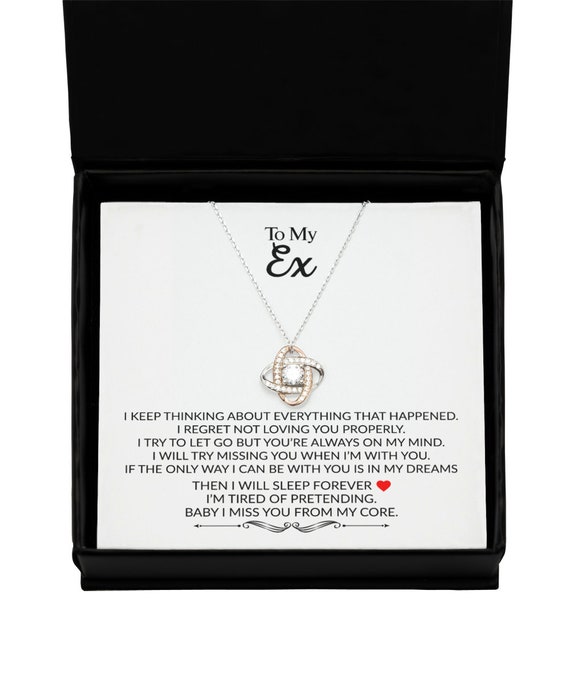The image depicts an open black jewelry box containing a heartfelt gift to an ex-lover. Inside the box, a white card prominently displays the heading "To My Ex." Suspended from the card is a delicate necklace with a thin silver chain, forming a V shape. The pendant features two interlocking ovals—one gold and one silver—embellished with small diamonds and intersecting in a swirly design. At the center of the ovals is a striking diamond-like stone.

Beneath the necklace, the card bears a poignant message: "I keep thinking about everything that happened. I regret not loving you properly. I try to let go, but you're always on my mind. I will try missing you when I'm with you. If the only way I can be with you is in my dreams, then I will sleep forever." The heartfelt text is accentuated with a red heart icon and an underscored line, conveying deep remorse and longing. This photograph captures the essence of a sentimental and romantic apology gift.